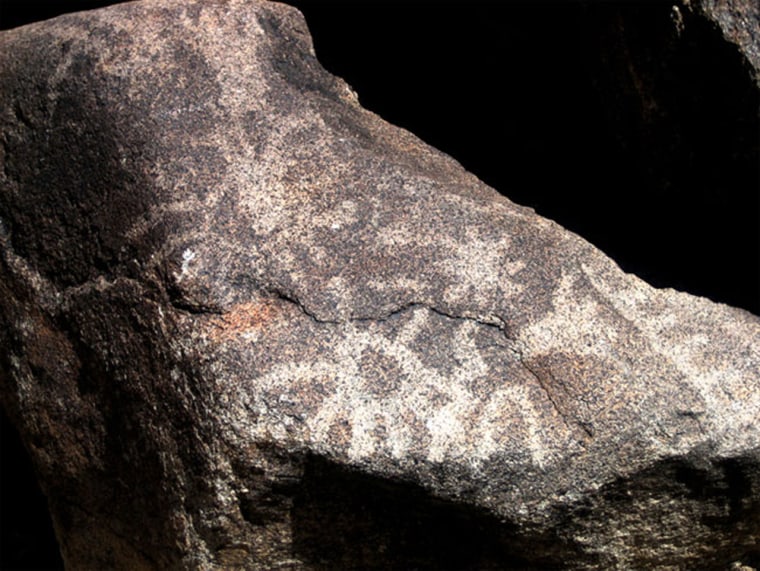The image shows a large, somewhat older-looking rock with a distinctive crack near its center and a predominantly darker coloration accented by various shades of black, grey, brown, and reddish-brown. Scattered across its surface are intriguing white markings resembling circles with radiating lines, reminiscent of crude sun or spider designs. The rock surface appears extensive enough to potentially accommodate a foot or two, giving it a sense of sturdiness that invites touch. Set against a uniform black background, the rock stands isolated, suggesting it could be photographed in a cave or on a black backdrop, emphasizing its rugged texture and the unusual, hand-drawn-like symbols adorning it.